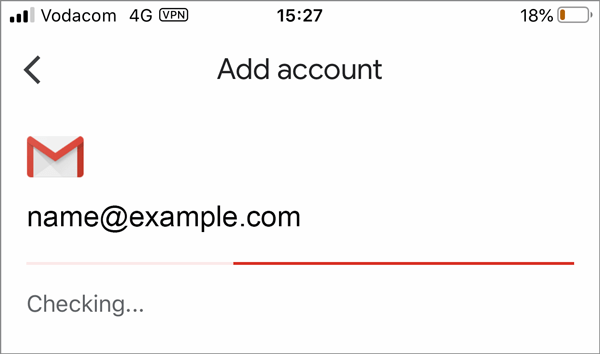The image displays a white box with a striking black border. In the upper left corner, three out of four signal bars are visible, accompanied by the text "Votacom 4G." Nearby, there's a rectangular box labeled "Rydat" followed by "VPN." Centered at the top of the image is the timestamp "15:27." On the top right, the battery icon is nearly empty, showing just 18% remaining.

Beneath this header section, a less-than symbol (<) appears on the left. In the central portion, the text "Add Account" is prominently displayed in large, black letters. Below this, to the left, is a red 'M' superimposed on an envelope icon. Adjacent to this icon is the black text "nameit@example.com."

Further down, a horizontal line spans the width of the image but stops short of reaching the edges. The left third of this line is pink, while the right two-thirds is a dark red. Below this line, on the lower left side, is gray text that reads "Checking..." The rest of the box contains ample empty space.